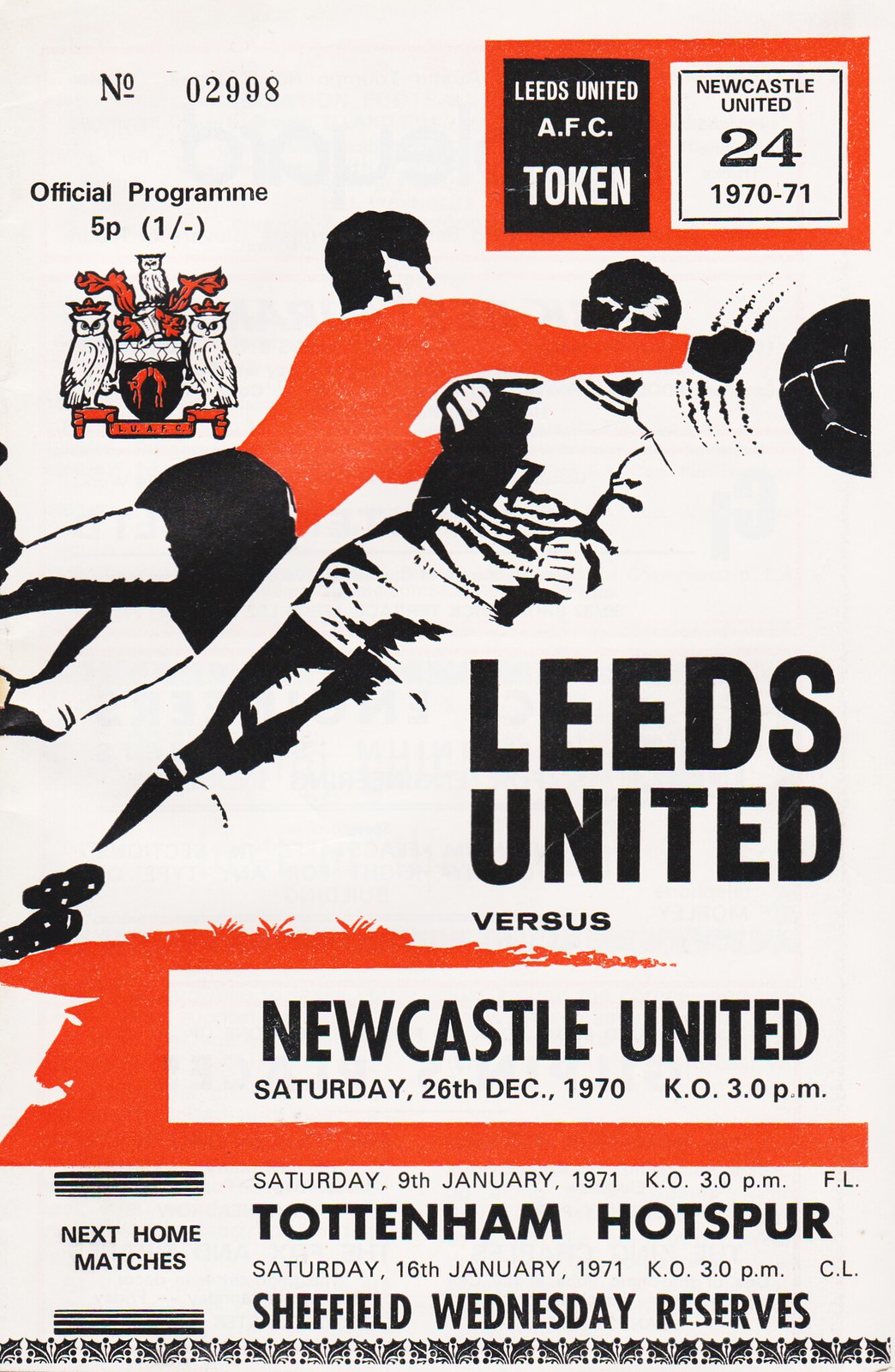This captivating vintage soccer program from December 26, 1970, features an exciting match between Leeds United and Newcastle United. The cover, marked as number 02998, prominently showcases an artistic illustration: a two-toned composition with one player in an orange top and black shorts, and another in monochrome. This dual-color layout, often considered challenging, adds a unique visual appeal. The program announces the match date and time—3:00 PM, alongside details for upcoming home games against Tottenham Hotspur on January 9, 1971, and Sheffield Wednesday Reserves on January 16, 1971. Additionally, there's mention of the Newcastle United's 1970-71 season in the top corner, emphasizing its historical significance. The booklet, priced at five pence, captures the essence of football heritage, making it a nostalgic artifact for fans. The details of the illustration, including a figure with long claw-like scratches across his back, add an intriguing, almost mysterious element to the artwork.